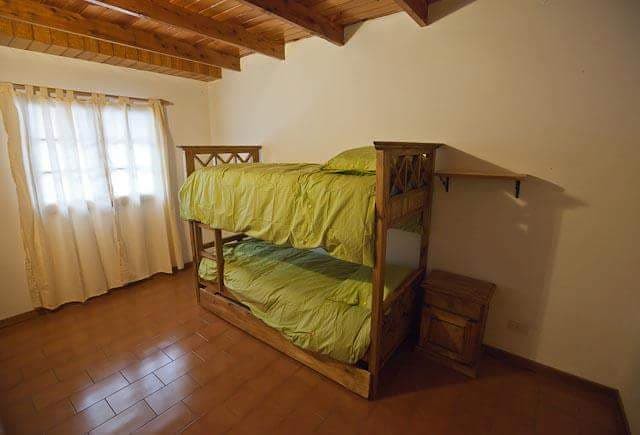This detailed photo of a bedroom captures a cozy and rustic aesthetic. The room features off-white walls and a wooden ceiling adorned with beams running across. The floor is wooden, arranged in a brick pattern, and it is a dark brown color. Dominating the room is a wooden bunk bed positioned against the wall, with wooden ladders on the left side. Both bunks are dressed with green blankets and matching pillows. To the right of the bunk bed is a nightstand, designed with a square lower cabinet and a rectangular pull-out drawer above it. Hovering above the nightstand is a wooden shelf supported by black hardware. Near the left side of the bunk bed, there is a standard window fitted with white sheer curtains that reach down to the floor, allowing soft, diffused light to filter into the room. The overall ambiance is one of warmth and subtle elegance, blending natural materials and serene colors.